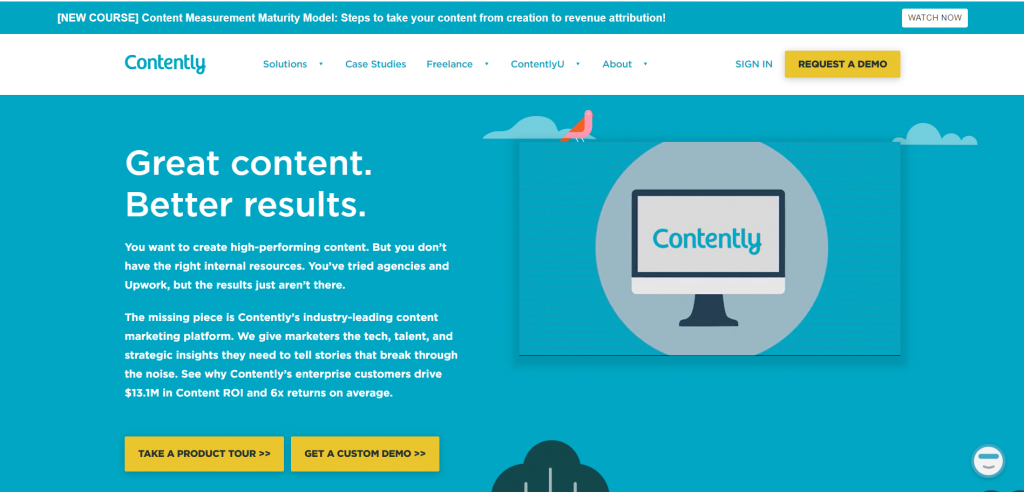This screenshot features a visually engaging website primarily dominated by a blue background. At the top of the page, there is a white, elongated rectangular banner housing a navigation bar with blue text. From left to right, the navigation links read: "Contently," "Solutions," "Case Studies," "Freelance," "Contently You," and "About." At the far right, the words "SIGN IN" appear in capital letters. Adjacent to this is a prominent yellow rectangular button with black text that says "Request a Demo."

Centered on the blue background, bold white text reads, "Great Content," followed by "Better Results." Below this, a paragraph in white text outlines the challenges of creating high-performing content: "You want to create high-performing content but you don't have the right internal resources. You've tried agencies and Upwork but the results just aren't there." Further down, the text affirms, "The missing piece is Contently's industry-leading content marketing platform. We give marketers the tech, talent, and strategic insights they need to tell stories that break through the noise. See why Contently's enterprise customers drive 13.1 million dollars in content and 6x returns on average."

Beneath this narrative, two yellow buttons with black text are displayed side by side. The button on the left invites users to "Take a Product Tour," while the one on the right encourages them to "Get a Custom Demo." On the far right of this section, a blue box showcases a black computer with a white screen, displaying the word "Contently" in blue text at its center.